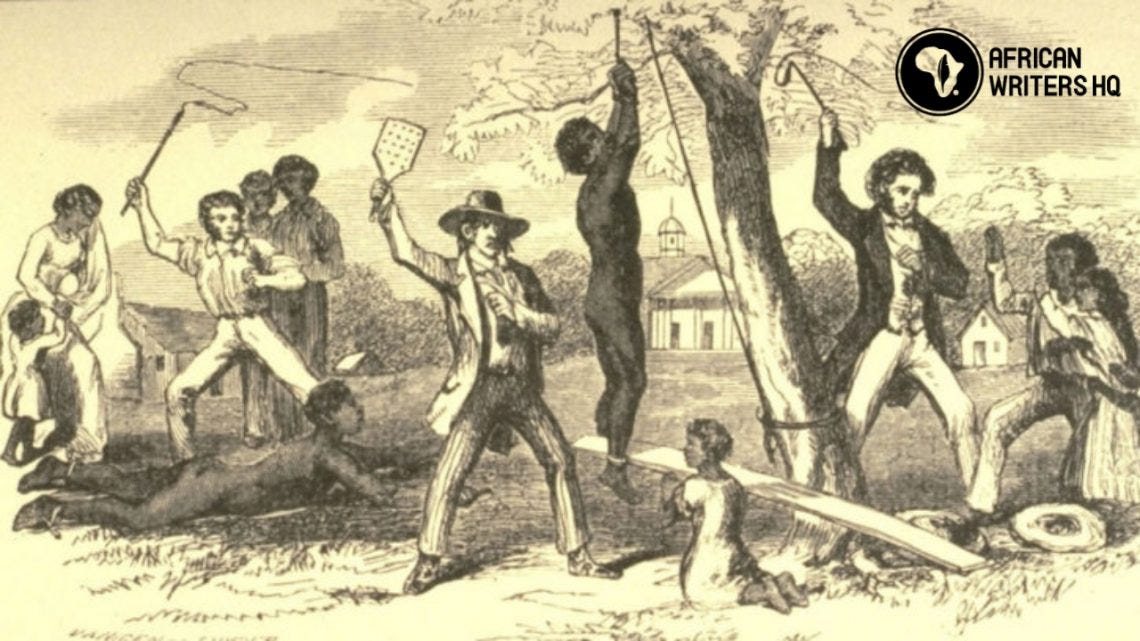This black and white historical engraving prominently titled "African Writers HQ" in the upper right-hand corner depicts a haunting and sorrowful scene of severe punishment and cruelty. At the very center, a large tree serves as a grim focal point, from which a naked black man is hanging by his wrists, his feet barely touching a board at the base. Kneeling at his feet is a young black woman in a dress, looking up at him. To the left of this ghastly scene, a white man wearing a cowboy hat and long, tapered coat, holds a square paddle, poised as if ready to strike. Further left, another black man lies face down on the ground while a white man stands above him brandishing a whip, its tail menacingly hanging in the air. On the right side of the engraving, a black man stands protectively, holding a young black girl, with his right hand raised defensively as if pleading for mercy. Towering over them is a white man with curly hair, his whip also raised, ready to rain down punishment. All the white men in the scene are featured wearing long coats and holding different instruments of torment. The backdrop of the engraving shows the continent of Africa inscribed within a circle, underscoring the tragic historical context of the brutalities exhibited in the image.